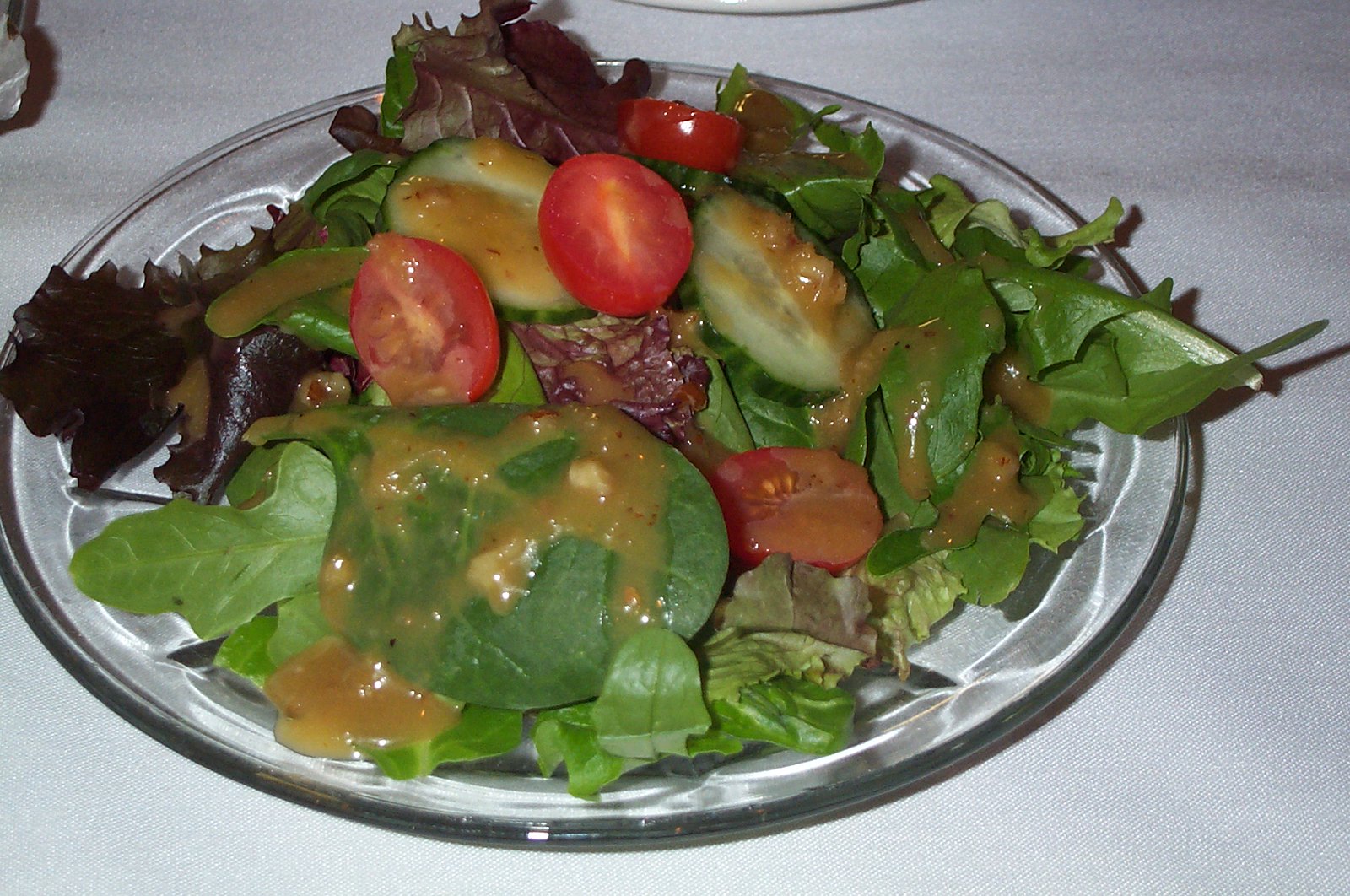The snapshot captures a salad arranged on a clear glass plate, which rests on a pristine white tablecloth in an indoor setting, possibly a home or restaurant. The photographic style of the image accentuates the details of the fresh vegetables in the salad. The salad features an appetizing mix of green lettuce leaves and darker red leaves, paired with baby greens and spinach for variety. It also includes vibrant cherry tomatoes sliced in half and two thick, unpeeled cucumber medallions. Generously drizzled over the vegetables is a bright orange dressing that resembles French or Italian vinaigrette. The absence of utensils in the photo keeps the focus entirely on the colorful, fresh salad atop its elegant plate.